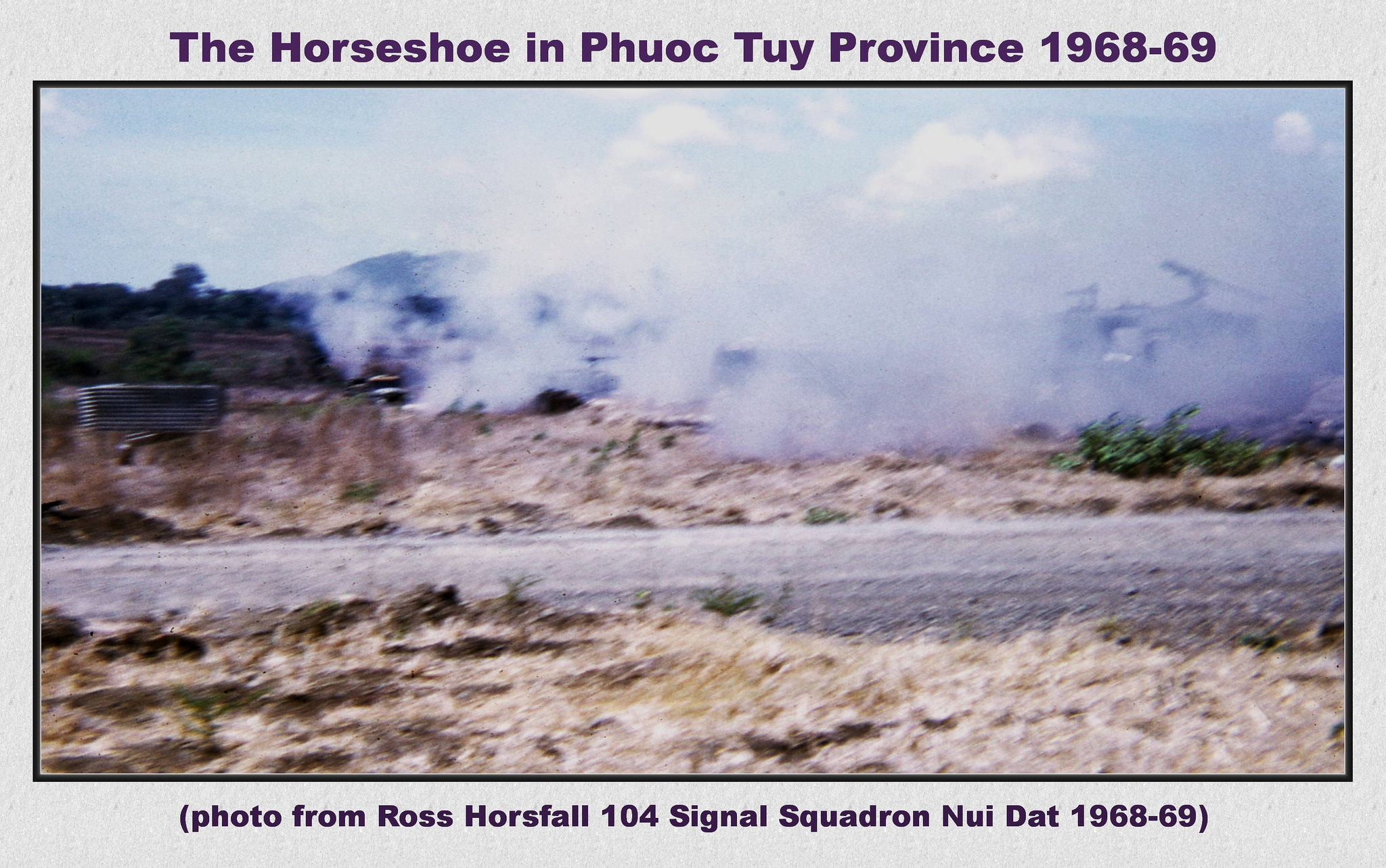The image captures a historical scene in Phuoc Thuy Province, 1968-69. Central to the photograph is a road stretching horizontally across the frame, surrounded by yellow dirt and dried brush. In the distance, thick smoke rises, obscuring much of the background and giving the impression of clouds on the ground, possibly from a fire. Faintly visible through the smoke is a vehicle on the right side, and far in the distance, one can discern hills and mountains to the left. The photograph is bordered in gray, with a caption in dark purple text at the top reading, "The Horseshoe in Phuoc Thuy Province, 1968-69." Below the photo, additional text in purple parentheses credits the photograph to Ross Horsefall of the 104 Signal Squadron, Nui Dat, 1968-69.